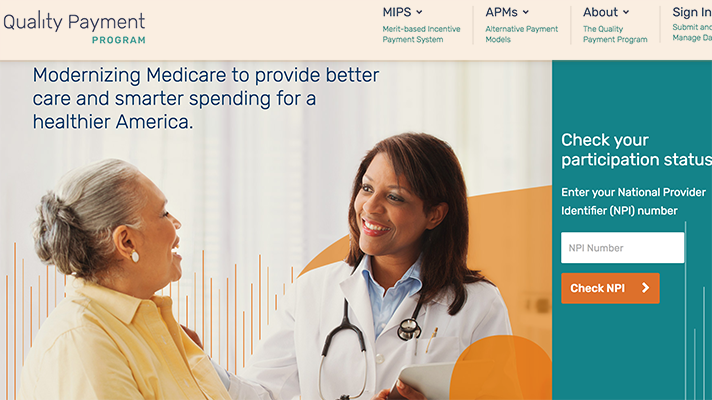The website features a sophisticated and informative layout designed for the Quality Payment Program. At the top, a beige banner prominently displays "Quality Payment Program" on the left side. "Quality Payment" is printed in a larger, thinner font with capitalized "Q" and "P", while "Program" is written in seafoam green, darker and capitalized, stretching from the "Y" to the "T" of "Payment".

Moving towards the center-right, there are several options with drop-down menus, including "MIPS" (Merit-Based Incentive Payment System), "APMs" (Alternative Payment Models), "About the Quality Payment Program," and "Sign-In, Submit and Manage Data".

Beneath this section is a graphic accompanied by a heading that reads, "Modernizing Medicare to provide better care and smarter spending for a healthier America," depicting a doctor and a patient in conversation.

To the right, there is a teal banner with white text stating, "Check Your Participation Status." Below this, instructions guide users to enter their National Provider Identifier (NPI) number into the provided space. An orange button labeled "Check NPI," with an accompanying right arrow in white text, allows users to proceed with their inquiry.